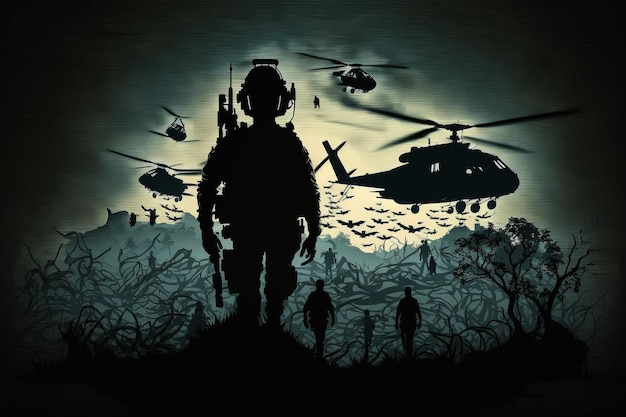In the center of a dark, possibly jungle landscape, illuminated by light, stands a silhouette of a heavily equipped army soldier. His figure is detailed with a large gun on his back, a helmet, and extensive gear, indicating readiness for battle. Surrounding him are smaller silhouetted army men, less detailed but clearly following his lead. The backdrop is dense with trees, branches, and foliage, creating an entangled scene that hints at a jungle environment, possibly reminiscent of the Vietnam War. Above, the sky is filled with dark clouds and a mix of silhouetted and somewhat illuminated helicopters, totaling four, flying at varying distances. The light from the helicopters cuts through the darkness, adding a dramatic effect. Additionally, there appear to be bats flying amidst the scene, adding a layer of eerie complexity. The entire scene appears to blend elements of a photograph and a painting, giving it a slightly surreal, shadowy, and flat dimensional feel.